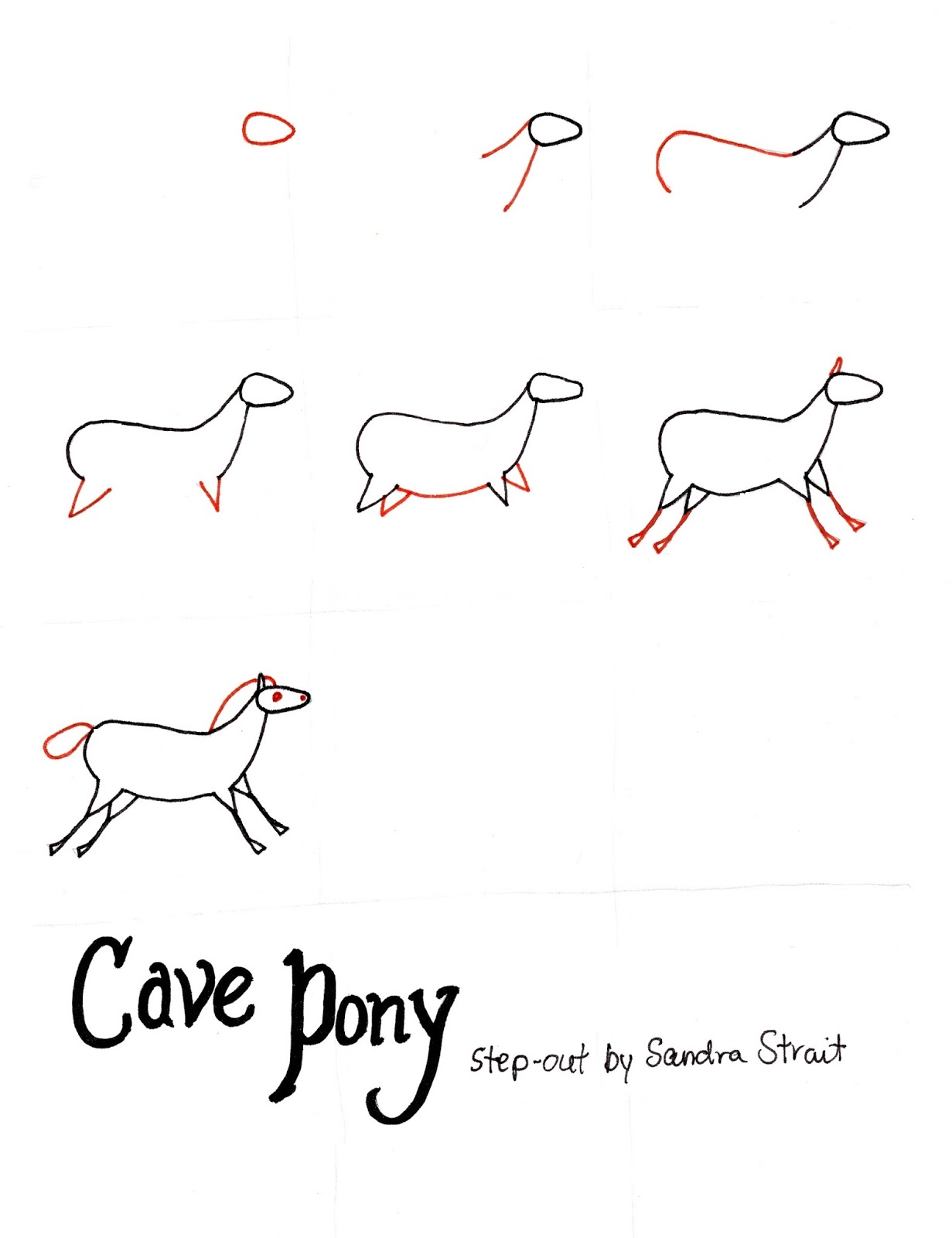The image is a detailed step-by-step guide on how to draw a cave pony by Sandra Strait, comprising seven stages. The first image presents a red circular shape, symbolizing the pony's head. In the second image, brown lines extend from the circle, forming the neck. The third illustration introduces another brown line outlining the body. The fourth step adds the legs, and the fifth step completes the underbelly and additional legs. The sixth image details the ears, hooves, and the final touches on the legs. The last image showcases the fully drawn pony, complete with its mane, tail, eyes, and mouth, resembling prehistoric cave art. The simple and instructional design, labeled "Cave Pony Step Out by Sandra Strait," provides clear visual guidance for sketching a cave pony.